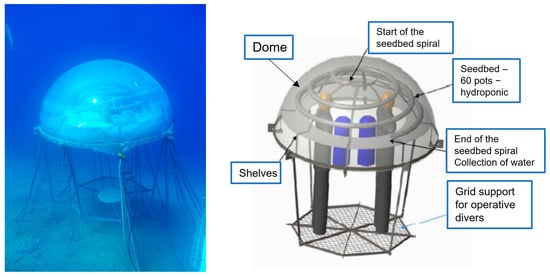This image depicts an underwater hydroponic farm consisting of a two-part illustration, with a photograph on the left and a detailed diagram on the right. The photograph shows a deep dark blue ocean floor, where a glass-topped dome structure is anchored by various cables and metal legs extending down to the seabed, securing it firmly in place. The water surrounding the dome is thick and crystal blue, making fine details challenging to discern.

On the right side, the diagram, rendered in gray, provides a comprehensive breakdown of the components of the dome. Clearly labeled, it identifies elements such as the 'dome,' 'shelves,' and 'grid support for operative divers' at the base. The dome serves as an underwater farm, beginning with the 'start of the seedbed spiral' containing '60 pots for hydroponics' and concluding with the 'end of the seedbed spiral' and a 'collection of water.' This setup appears to facilitate the growing of plants beneath the ocean's surface, with provisions for divers to conduct maintenance intimately described in great detail.